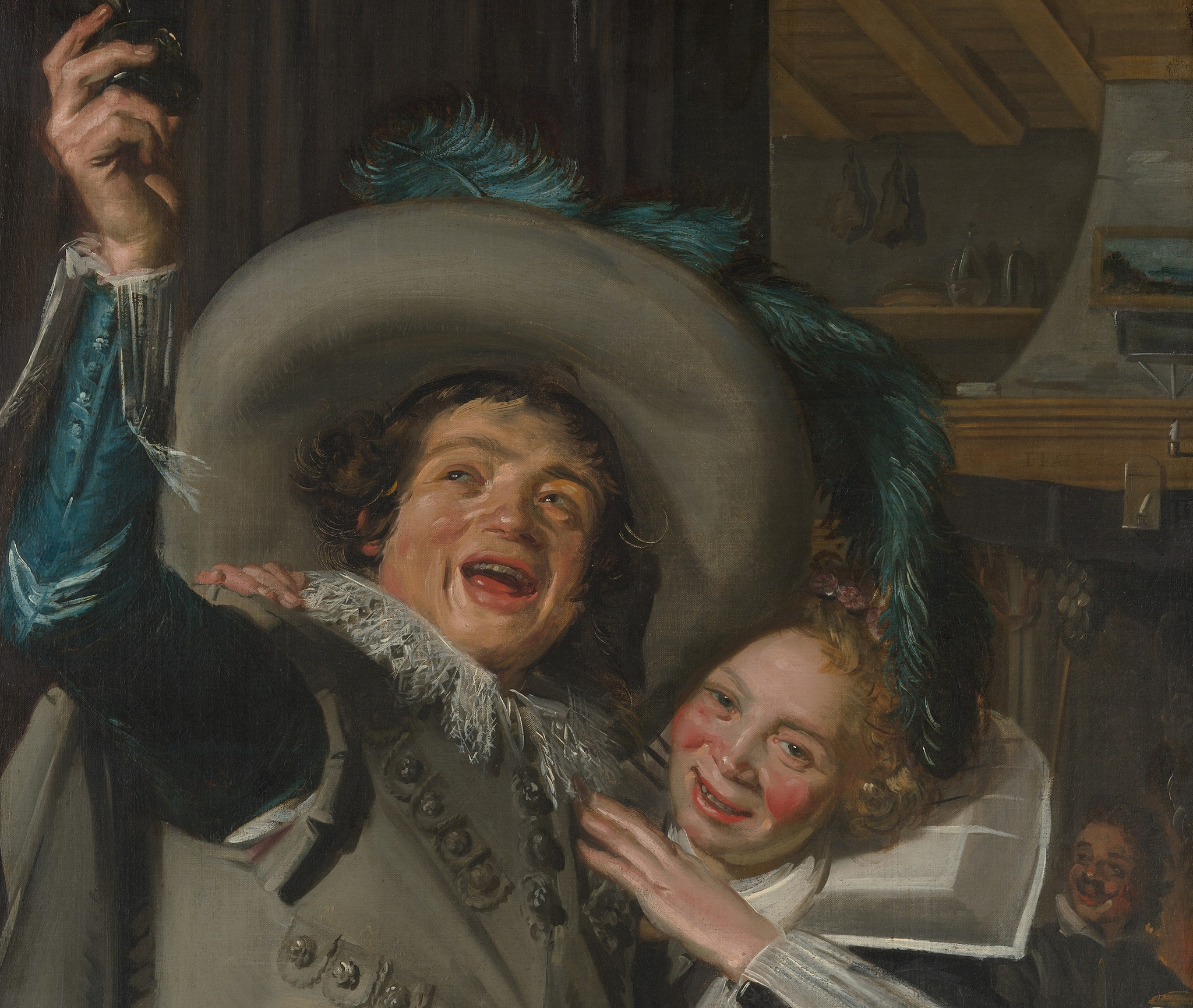This detailed painting captures the lively scene of two jubilant figures in the ambiance of a vintage pub, characterized by intricate interior woodwork and quaint wall paintings. The central figure, a young boy, commands attention with his festive large green hat adorned with blue feathers, a flamboyant Victorian-style collar, and a coat with dark buttons over a blue shirt with turquoise fringed sleeves. He holds a glass of brandy or cognac aloft, his face lit with a joyful expression. Beside him stands a girl with curly blonde hair, her cheeks flushed red with merriment. She mirrors his Victorian collar, though hers is more ornate, over a white shirt. Both figures exude happiness, highlighting their spirited camaraderie. Behind them, another man grins widely, augmenting the spirited atmosphere. The scene is further enriched by a shelf with various trinkets, adding to the pub's charmingly rustic décor.